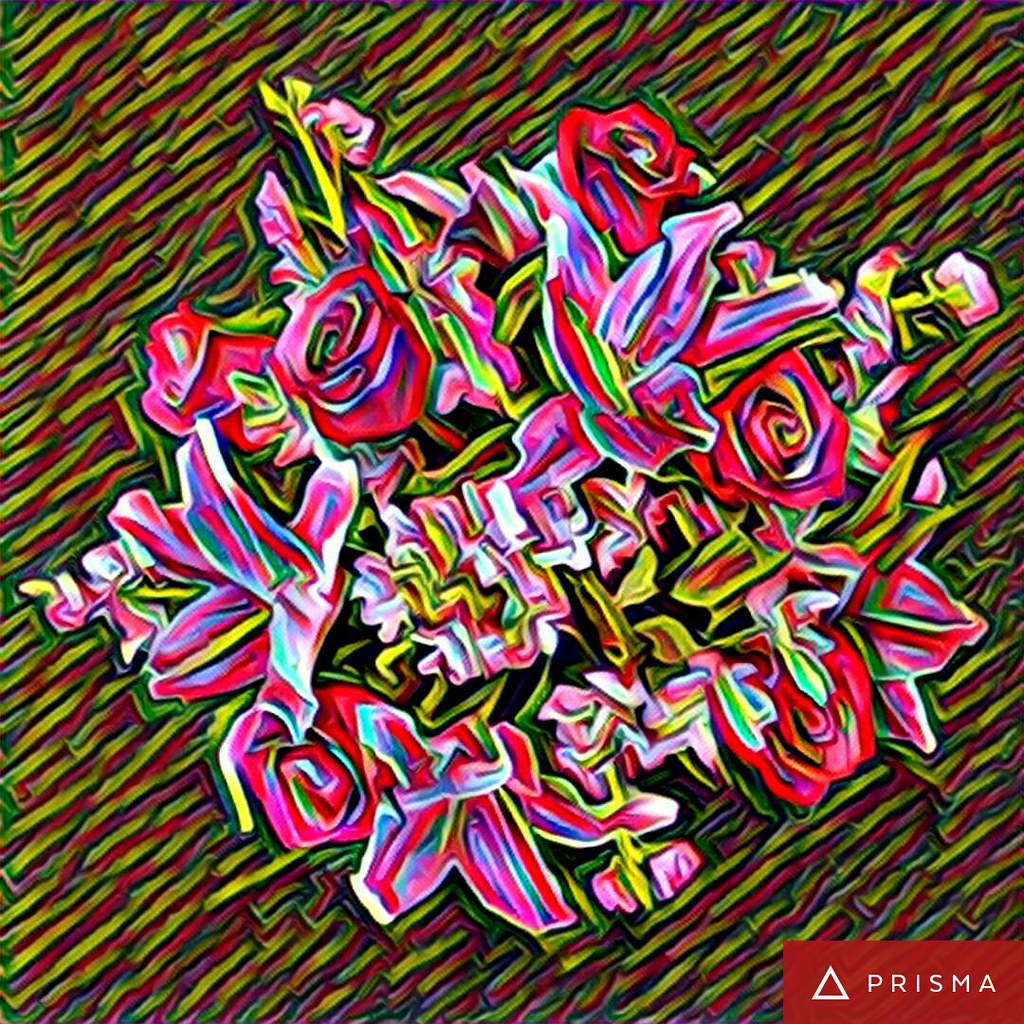The image presents a vibrant, abstract illustration, likely AI-generated, that features a striking bouquet of roses in red, pink, and hot pink hues. These roses, detailed with green petals and blossoming buds, create a captivating, almost digitalized effect with a glitch-like quality. The roses stand out vividly against a dynamic background of diagonal stripes colored in green, red, yellow, and blue. The background also exhibits a darker, wavy, oil painting texture that complements the flower bouquet. Adding to its artistic flair, the image includes a watermark in the bottom right corner, consisting of a red rectangle with a white triangle inside it and the word "Prisma" capitalized next to it, indicating its creation using the Prisma app.